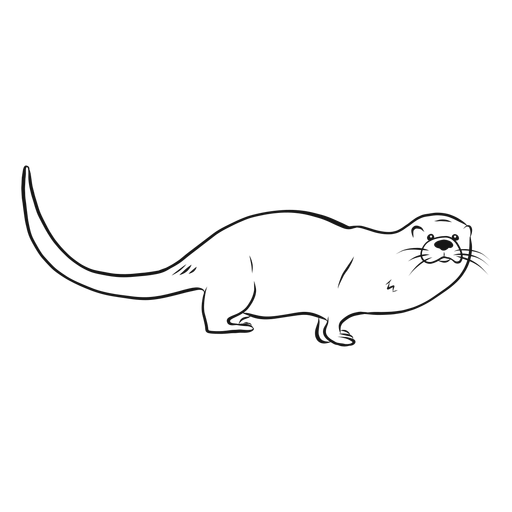A simple, black-and-white line drawing depicts an otter standing on all four legs, its long tail elevated. The image focuses solely on the otter, set against an entirely white background. The illustration, while not rich in intricate details, clearly outlines the otter's main features: it has small, beady eyes, a prominent black nose, and whiskers extending from either side of its mouth. Its two ears, paws, and legs are minimally detailed. The otter is centrally positioned, facing the viewer directly, giving a straightforward view of its facial features and body stance.